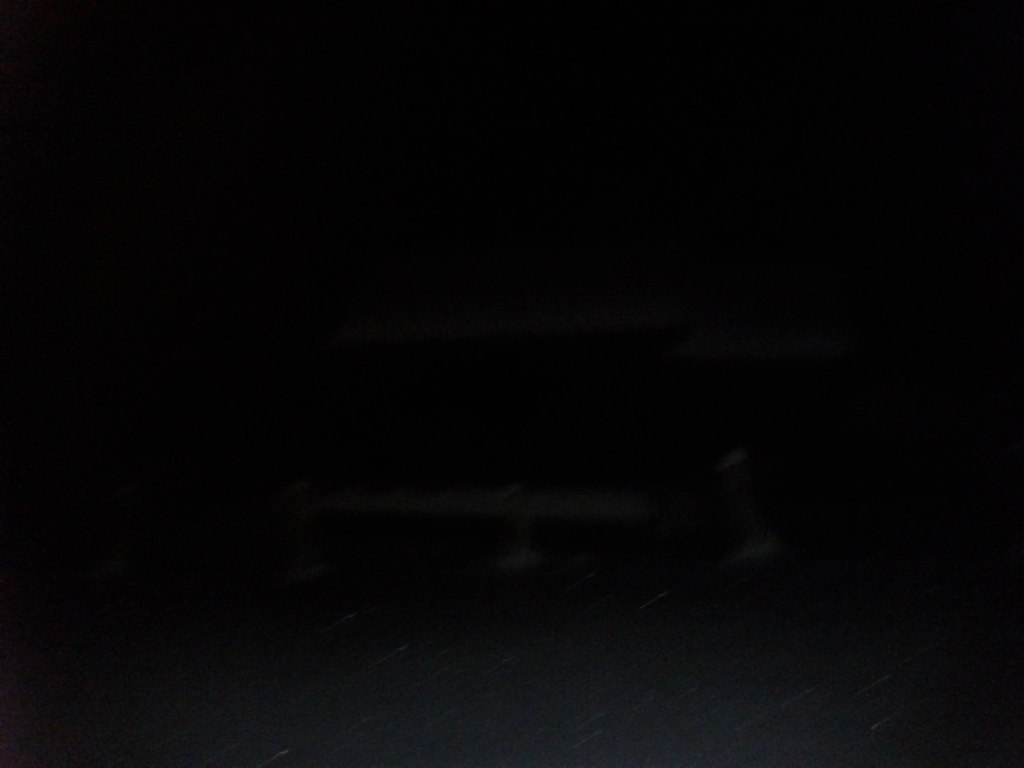In this nighttime photograph, the scene is predominantly dark, creating a stark contrast with several key elements illuminated by the camera flash or ambient light. In the upper portion of the image, we see the edge of a roof coated in a layer of white snow, which adds a crisp, reflective quality to the otherwise shadowed backdrop. Below the roof, part of a wooden fence is visible, adorned with patches of snow clinging to its surface, emphasizing its texture. Towards the bottom quarter of the picture, a light gray area emerges, likely the snow-covered ground, interspersed with streaks of white snow. On both the left and right sides of the fence, wooden stumps protrude, also dusted with snow at their bases and tops, further adding to the scene's wintery atmosphere. This meticulous snowfall on various elements—the roof, fence, and stumps—creates a serene, chilly nighttime landscape.